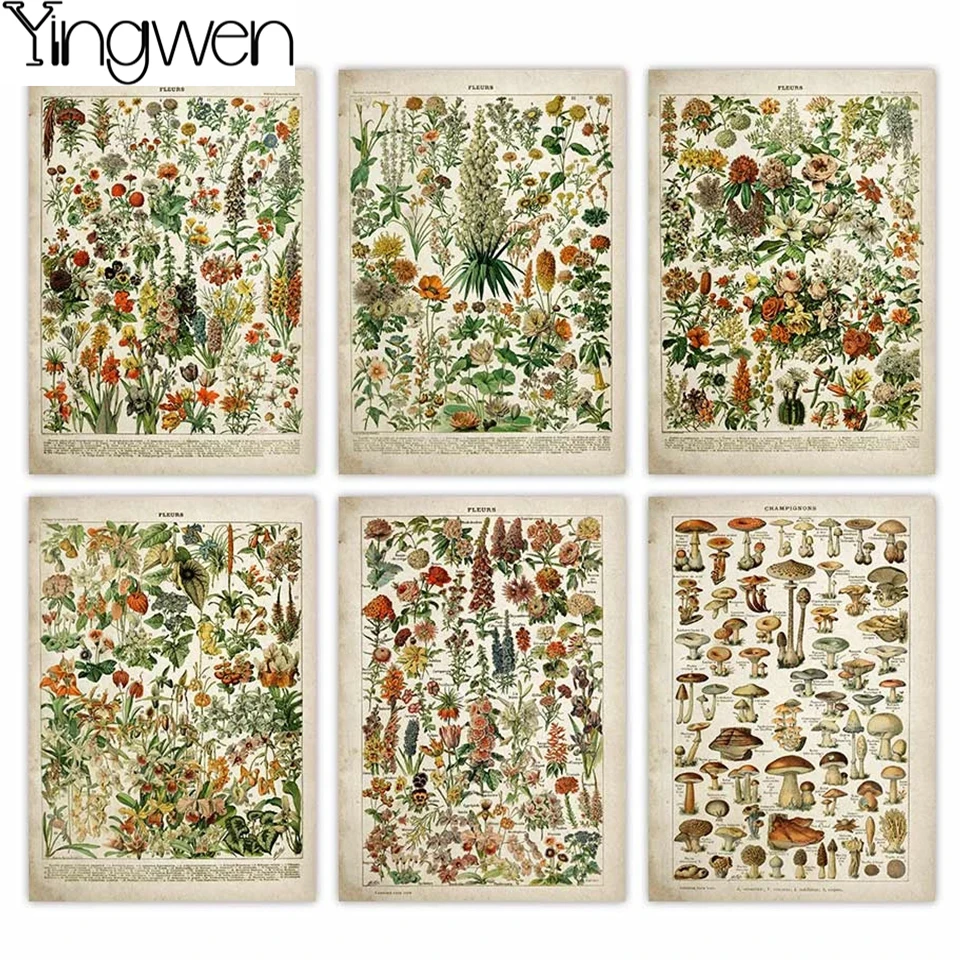The image depicts a collection of six vertical, rectangular posters arranged in two rows and three columns. Each poster showcases intricate illustrations of various plants and flowers, reminiscent of botanical book pages. The posters have a cream-colored background with worn, brownish-tinted edges, giving them a vintage appearance. The artist's name, Ying Wen, is prominently displayed in the top left-hand corner of the first poster, written in capital letters: Y-I-N-G-W-E-N. The top row features a range of floral illustrations with predominant red and pink hues, as well as green foliage. The first poster is slightly shorter than the others. The bottom row continues the botanical theme with different types of leaves and flowers, including cone-like blooms. However, the last poster in the bottom right corner stands out by displaying various mushrooms and fungi, adding a unique element to the set. Overall, despite the individual differences in plant types and colors, the posters maintain a cohesive and harmonious aesthetic.